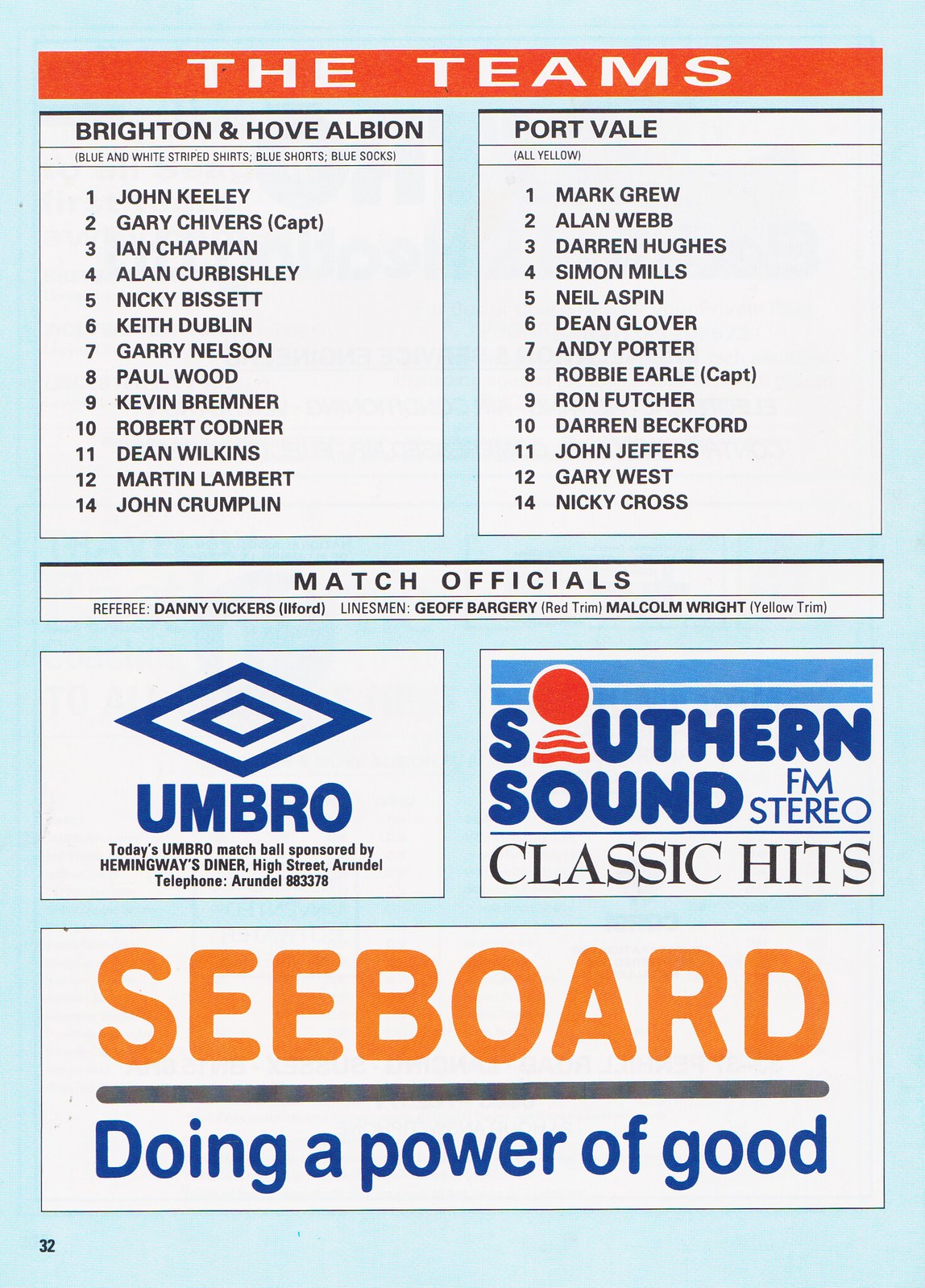This image features a detailed pamphlet for an English soccer game. At the top, set against an orange background, the teams are listed in white text. On the left side, the roster for Brighton and Hove Albion is displayed, enumerating players 1 through 14. Opposite, on the right, is the lineup for Port Vale, similarly listing players 1 through 14. Below these lists, the pamphlet details the match officials, including referees, linesmen, and specifically mentions Malcolm Wright. Further down are several advertisements: on the left, an ad for Umbro featuring blue text and their signature triangle symbols; to the right, an ad for Southern Sound FM Stereo Classic Hits, where the 'O' in 'Southern' is stylized as a red circle with a half-circle beneath it. At the bottom, there is an ad with 'Seaboard' in orange text and 'Doing a Power of Good' in blue text.